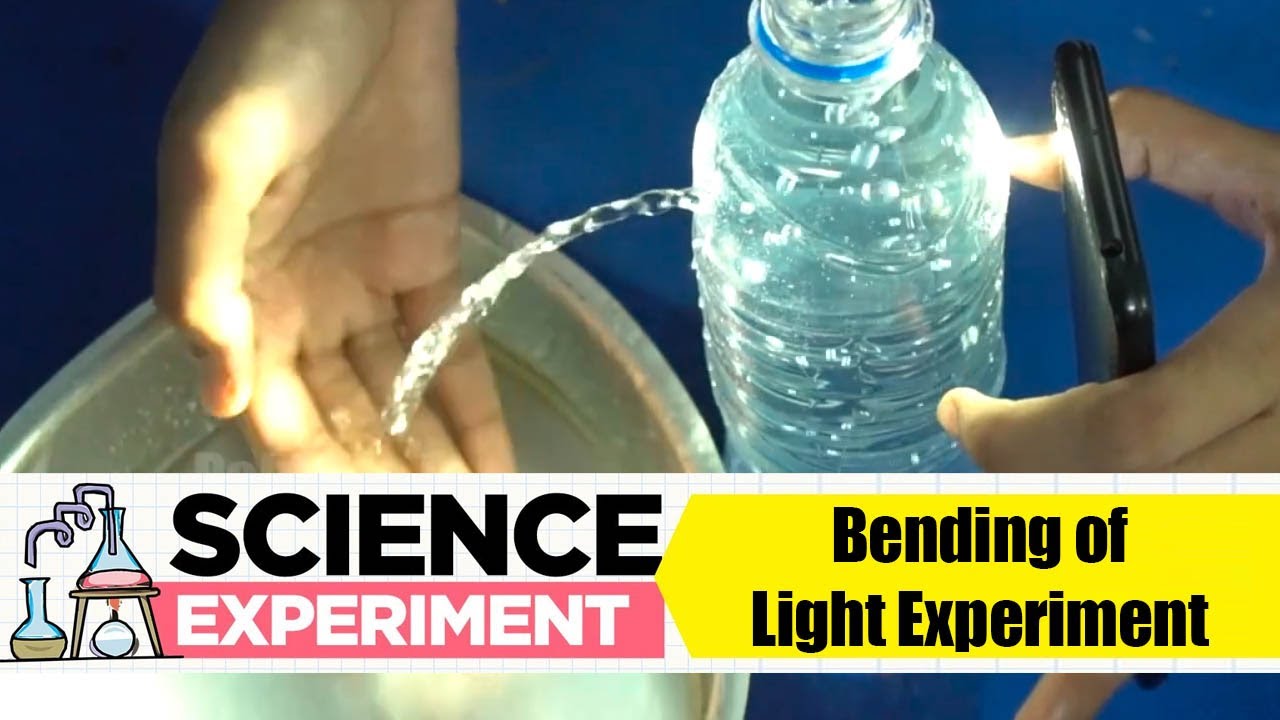The image depicts a detailed science experiment labeled "Science Experiment" and "Bending of Light Experiment." Set against a blue background, the scene features a clear water bottle with a blue cap, punctured on one side, causing water to leak out. A person’s right hand catches the leaking water, while their left hand holds a black cell phone with its flashlight turned on, shining directly into the bottle. The light from the phone illuminates the water stream, highlighting the effect of light bending through the falling water. Additionally, a metal bucket is visible in the bottom left corner. At the bottom of the image, a white bar contains large black text reading "Science" and smaller white text over a pink background reading "Experiment." On the right, a yellow bar with bold black lettering reads "Bending of Light Experiment." The image is bright, with a clear, sharp quality, and includes a cartoon test tube on the left side of the text bar.